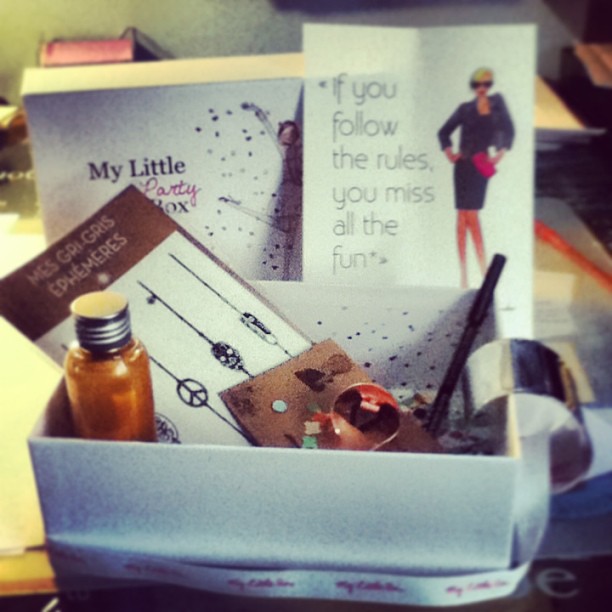The image features a neatly arranged white box adorned with a ribbon, containing a variety of items primarily used by females. Inside the box, there is a brown vial and a booklet with a brown and white cover, as well as some homemade arts and crafts pieces. One of the papers inside displays the text "MESGRIGRISFMERSEPHEMERES" in different languages, surrounded by white and black symbols, one resembling a skull. Propped behind the box are two distinct cards: one features a graphic of a blonde woman in a black outfit and skirt, holding a pink clutch with the quote, "If you follow the rules, you miss all the fun." The other card shows a person dancing and partially reads "My Little Party Box." The background is slightly out of focus, emphasizing the main colors of white, pink, and brown throughout the image.